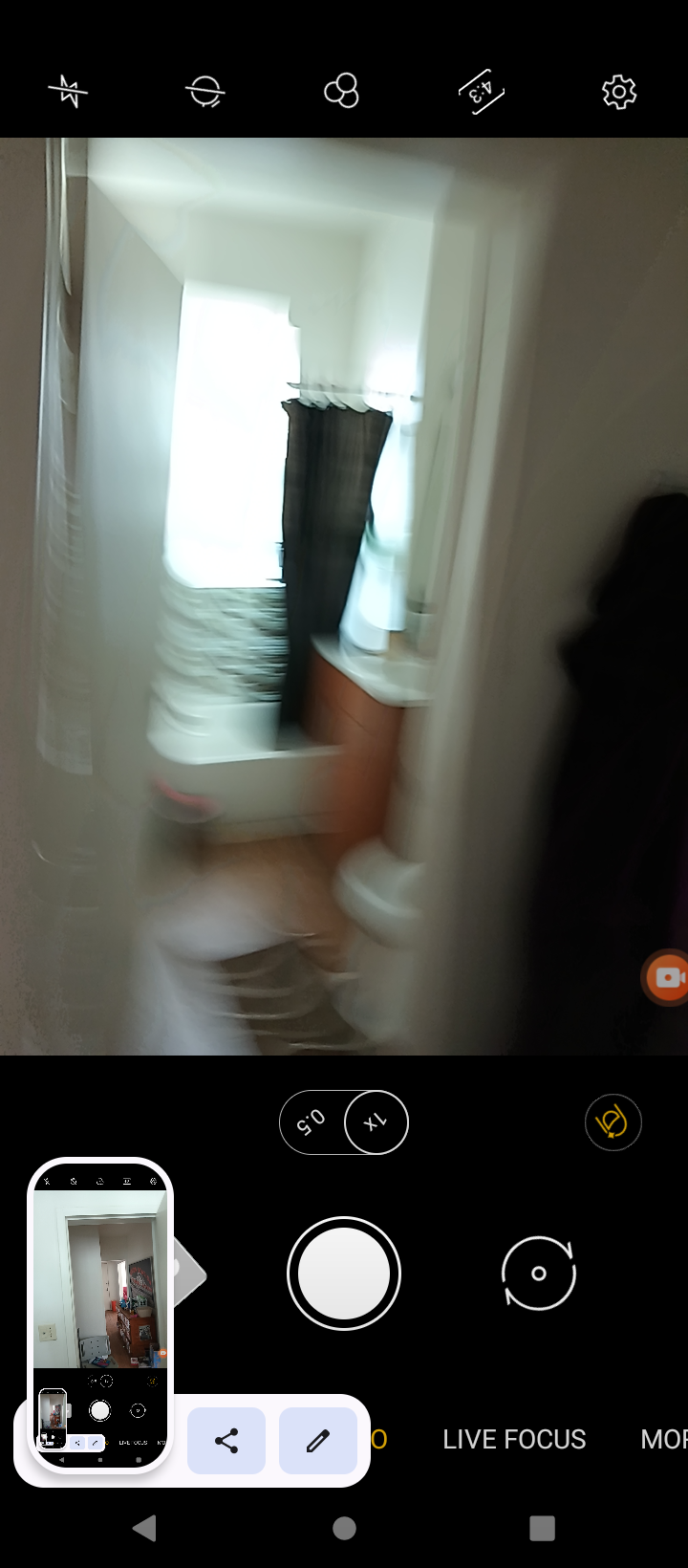The image captures a video being recorded on a smartphone, evident from the black bars at the top and bottom of the screen and the various control buttons typically found on a recording interface. The scene portrays a blurry view of a bathroom. The bathroom features an open white door, beyond which hangs a black shower curtain over a white bathtub. A window is situated within the bathing area, allowing a slight touch of natural light. The vanity unit is brown with a white countertop. Adjacent to it, the edge of a white toilet is partially visible. The perspective suggests the photographer is standing in a hallway, indicated by an assortment of clothes hanging on the wall to the right. Additionally, the bottom portion of the image shows the smartphone's interface for adjusting focus, taking pictures, viewing the last captured image, and other options.